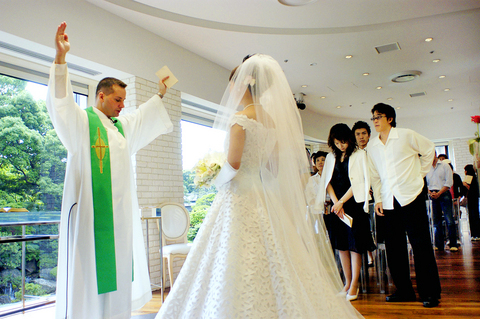In this indoor wedding ceremony, a young male priest with short brown hair and pink skin stands on a brown hardwood floor, beneath a white ceiling and surrounded by white walls, including a section of white brick. He is adorned in a full-length white robe complemented by a green sash featuring golden rhombuses with red crosses. The priest, clasping a piece of paper in his left hand, raises his hands, his head bowed and eyes closed in solemnity, as he performs the ritual in front of a bride. The bride, seen from the back, wears a short-sleeved gown that flares out elegantly and a long veil draped over her updo, adorned possibly with a white flower and pearls. The venue, adorned with a window that offers a view of lush green trees, is populated by attendees, including a woman and two men who appear to be of Asian descent, all standing solemnly. The groom is presumably present, though obscured by the bride's dress and the photo's angle. The serene atmosphere captures the solemnity and elegance of the occasion.